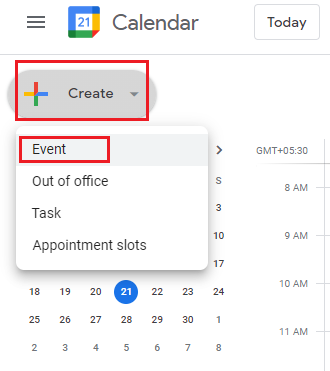This cropped image of the Google Calendar interface showcases the options available for creating an entry. At the top, there is a drop-down list menu. Below it, the Google Calendar logo appears next to the calendar title. To the right, today's current time is displayed. The image includes two red outlined squares, which are not part of Google Calendar's original design; these have been added to highlight the "Create" event button and a specific event itself.

Upon clicking the "Create" button, a pop-out window reveals four options: Event, Out of Office, Task, and Appointment slots. Behind this pop-out window, the calendar view is partially visible, specifically highlighting the 21st. The y-axis displays time slots ranging from 8 a.m. to 11 a.m., and the GMT time zone is indicated on the right. The background of the interface is white, and other elements of the webpage have been cropped out, focusing solely on the calendar interface.